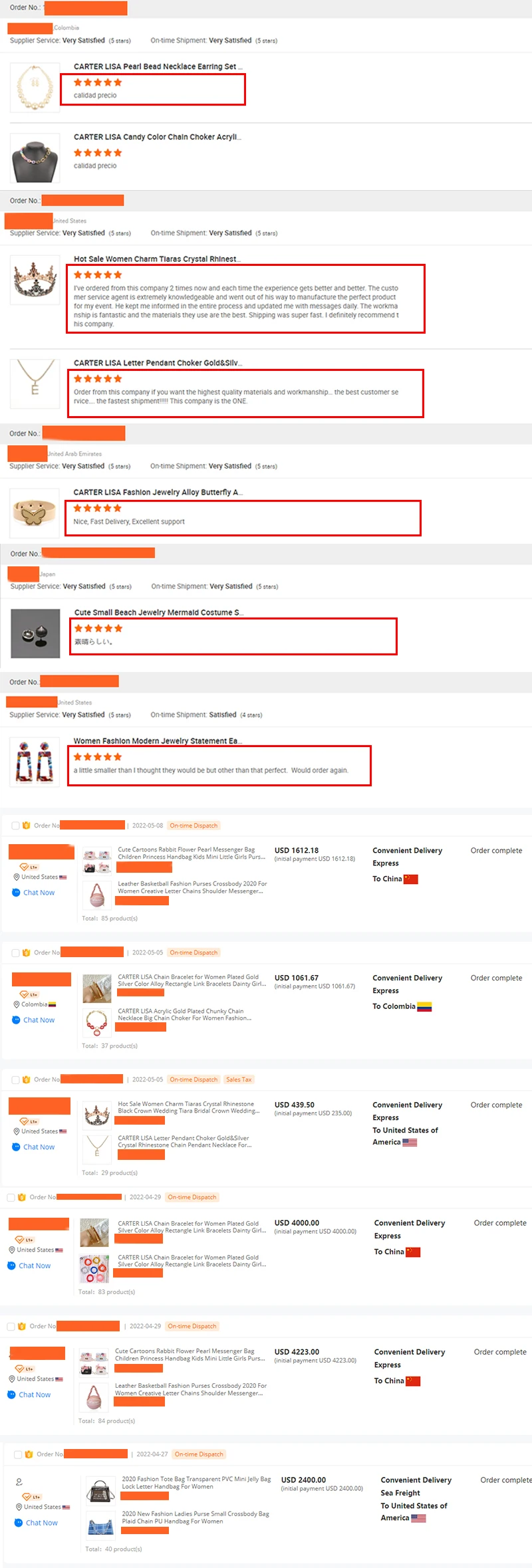This image portrays a page from a website dedicated to selling jewelry, primarily showcasing an array of necklaces. The page includes various styles and designs, interspersed with ratings prominently featuring numerous five-star reviews. The stars and certain highlights are marked in orange, drawing attention to customer feedback and ratings. Though the text is very small and illegible, the visual arrangement suggests that the page also includes user comments and descriptions of each necklace. There's a section with blue elements on the left side, likely representing clickable options or navigation tools, though their specifics are indistinct. The overall layout suggests a comprehensive online marketplace for jewelry, with features designed to help users evaluate and select pieces based on ratings and possibly reviews.